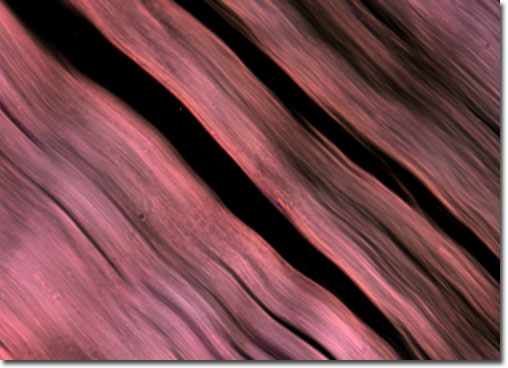The image is an enigmatic, artistic portrayal, possibly a photo or a drawing, characterized by a series of reddish-pink, striated, wavy strokes running diagonally from the top left to the bottom right. The composition features alternating sections of these reddish-pink waves and thick black lines, creating a visually striking contrast. The background is predominantly black, which further highlights the waves. The pattern is irregular, with variations and imperfections, including slight circles and dots, adding to the image's uncertain and intriguing nature. The overall dimensions of the image appear to be rectangular, despite its initial square-like impression.